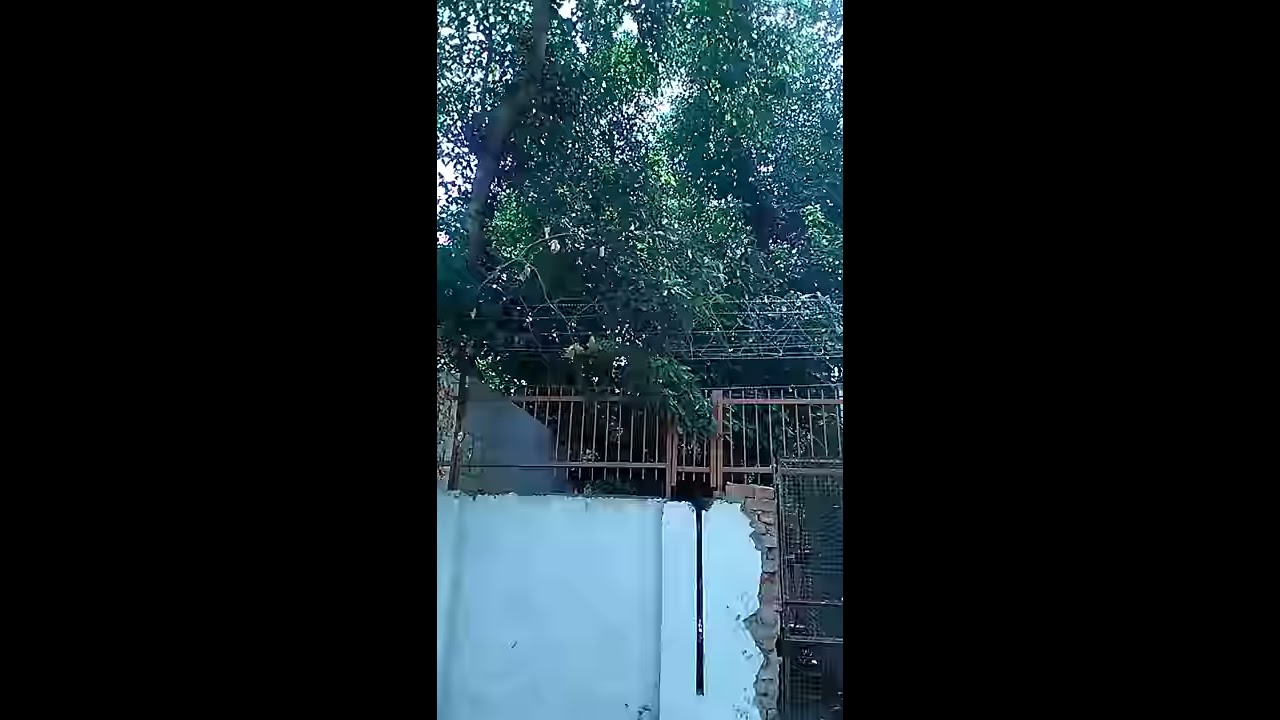The image is a vertical view of an outdoor scene framed by solid black bars on the left and right sides. In the center, there is a bright daytime sky with hints of blue and white clouds visible through a canopy of green leaves at the top. The foliage is dense, creating a natural border around the central features of the image. Dominating the middle section is a wrought iron fence, brownish-red in color, with vertical metal bars. This fence sits atop a white retaining wall made of concrete, although parts of the edge appear to be constructed from brick. Some of the tree branches and leaves hang over the fence, adding to the vegetation-rich atmosphere. The bottom of the wall, as well as further details, are cut off by the frame of the picture. The image is captured at a slight upward angle, emphasizing the towering trees and structural elements.